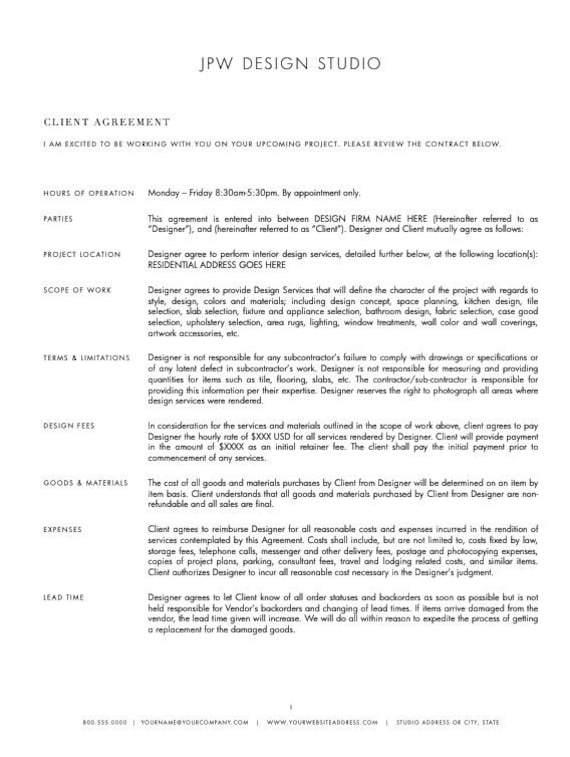This image is a detailed screenshot of a professionally formatted contract titled "JPW Design Studio Client Agreement". The heading at the top of the document clearly states the name of the design studio and the nature of the document. Following the heading, there is a welcoming note from the designer expressing excitement about the upcoming project and requesting the client to review the contract below.

The contract consists of several essential sections, each well-organized and clearly separated by titles for easy reference. The categories covered in the contract include **Hours of Operation** (Monday through Friday, 8:30 a.m. to 5:30 p.m. by appointment only), **Parties** (defining the agreement between the "designer" and the "client"), **Project Location**, **Scope of Work**, **Terms and Limitations**, **Design Fees**, **Goods and Materials**, **Expenses**, and **Lead Time**. Each section contains detailed information pertinent to establishing mutual understanding and agreement between the designer and the client.